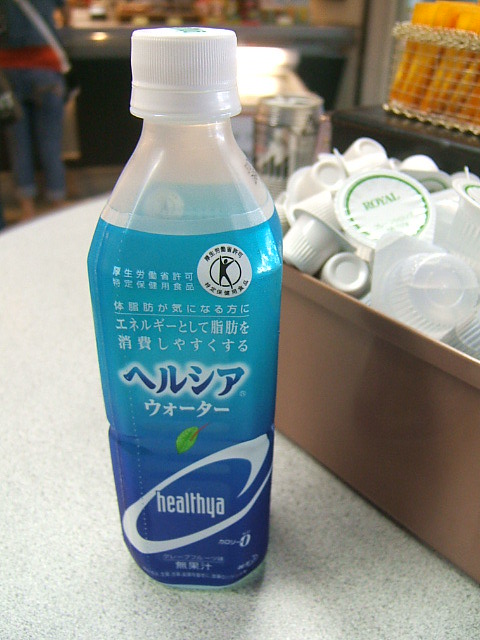The photograph captures a close-up of a plastic beverage bottle prominently displayed on a grayish formica counter inside what appears to be a Japanese store or a self-serve area in a convenience store. The plastic bottle, which holds a 12-ounce drink, features a two-tone blue label—light aqua blue at the top fading into a darker blue towards the bottom. The label is predominantly in Japanese characters, with the English word "Healthier" (or a variant of it like "Healthia" or "Healthqua") written at the bottom, accompanied by a swirl design. The bottle has a white cap, and its top section is partly transparent. To the right of the bottle, there’s a red plastic container filled with small, peel-off milk creamers, and nearby are some yellow self-serve spoons, hinting at a section where customers can prepare their drinks. In the blurred background, we can make out glass-fronted counters typical of areas where goods are selected and handed over by store personnel, and there's a person wearing rolled-up blue jeans and a gray shirt, adding to the bustling atmosphere of the store.